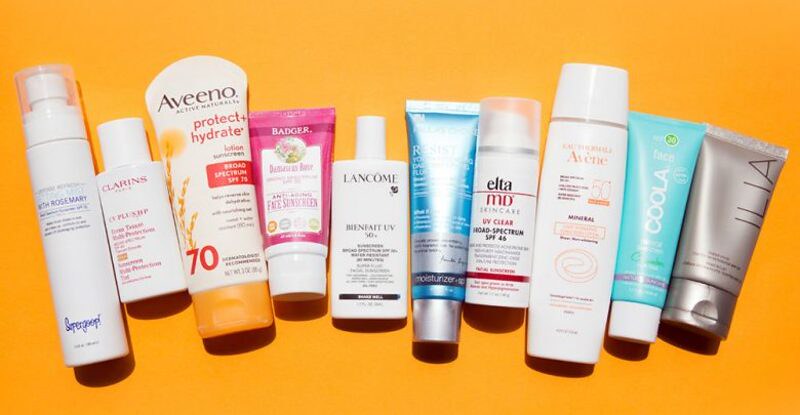An array of diverse cosmetic products is elegantly arranged on a vibrant yellow-orange background. From left to right, the lineup begins with a Supergoop Rosemary Spray, elegantly packaged in a white, round bottle capped with a clear top. Next, a diminutive Clarins bottle featuring red text and a sleek, opaque cap sits prominently. This is followed by an Aveeno Protect + Hydrate sunscreen, boasting a robust SPF 70 and adorned with a dandelion graphic at the base, complemented by a distinctive yellow seashell cap.

The fourth item in the lineup is a whimsical pink bottle from Badger, topped with an opaque cap and hinting at a floral essence. Following this is a medium-sized Lancôme bottle, pristine in white. Moving along, a mystery blue tube catches the eye; its reflective finish makes the brand name elusive, but "moisturizer" is prominently displayed in black and white letters on a silver label, and it is crowned with a silver cap.

Positioned thereafter is an EltaMD UV Clear Broad-Spectrum SPF 46, presented in a sleek spray bottle with a clear top and a signature red-striped label. An Aveeno product ensues, housed in a large squeeze bottle with an opaque top. The penultimate item is a Coola sunscreen, packaged in a refreshing mint green bottle with a white top. Finally, the collection concludes with an Ilia product, impeccably encased in a silver bottle with a matching silver cap, completing the assorted display of cosmetic essentials.